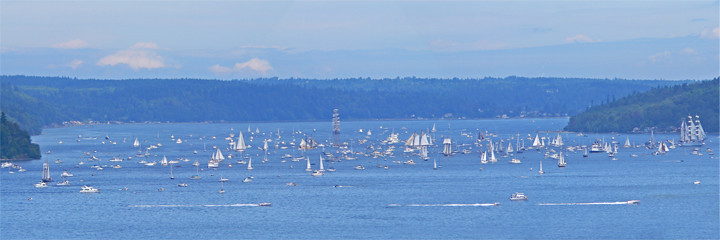The image presents a distant, wide-angle shot of a bustling waterway, likely a bay or a wide river, framed by green, forested land. The deep blue water extends into the horizon, curving slightly, creating a picturesque background with subtle mountainous terrain. The sky is a mix of blue and white, dotted with puffy clouds, adding a peaceful charm above the active scene below.

The water is teeming with marine activity, featuring a substantial number of small white sailboats, possibly numbering over a hundred. Among these, there are also larger sailboats with multiple decks and sails, creating a diverse flotilla. Some boats appear to be jet skis, though they are hard to distinguish due to the considerable distance and high vantage point from which the photo is taken. This multitude of boats cluster in the middle of the waterway, their white wakes casting long stripes across the blue surface, hinting at the liveliness and movement within this serene natural setting.